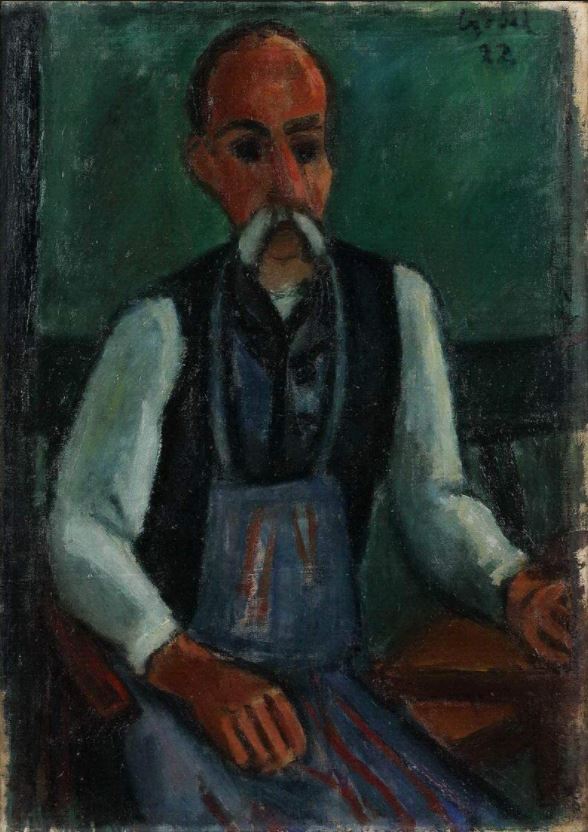This painting depicts an older man with distinctive features, prominently characterized by a large white handlebar mustache that droops on either side of his face. He has thinning dark hair with a noticeable receding hairline and dark eyebrows, complementing his peach-colored skin. He is dressed in a long-sleeved white shirt beneath a dark vest and wears a blue apron, which is adorned with red lines. The man is seated at a table, with his right hand resting on his knee and his left hand positioned on the table's edge. He exudes a neutral expression, looking straight ahead. His attire and demeanor suggest the possibility of a profession such as a cook, butcher, or bartender.

The background is a mix of light green and black shades, depicting what appears to be a wall. The brown chair he sits in features a dark black backrest, and the surface he rests his arms on is also brown. In the top right corner of the painting, an artist's signature is visible but partially illegible, possibly reading "Geo Godot" with numbers that seem to be either 12 or 22. The top section of the painting contains dark bluish hues resembling window reflections or additional strokes of paint. The medium used appears to be oil pastels, giving the artwork a thick, crayon-like texture.